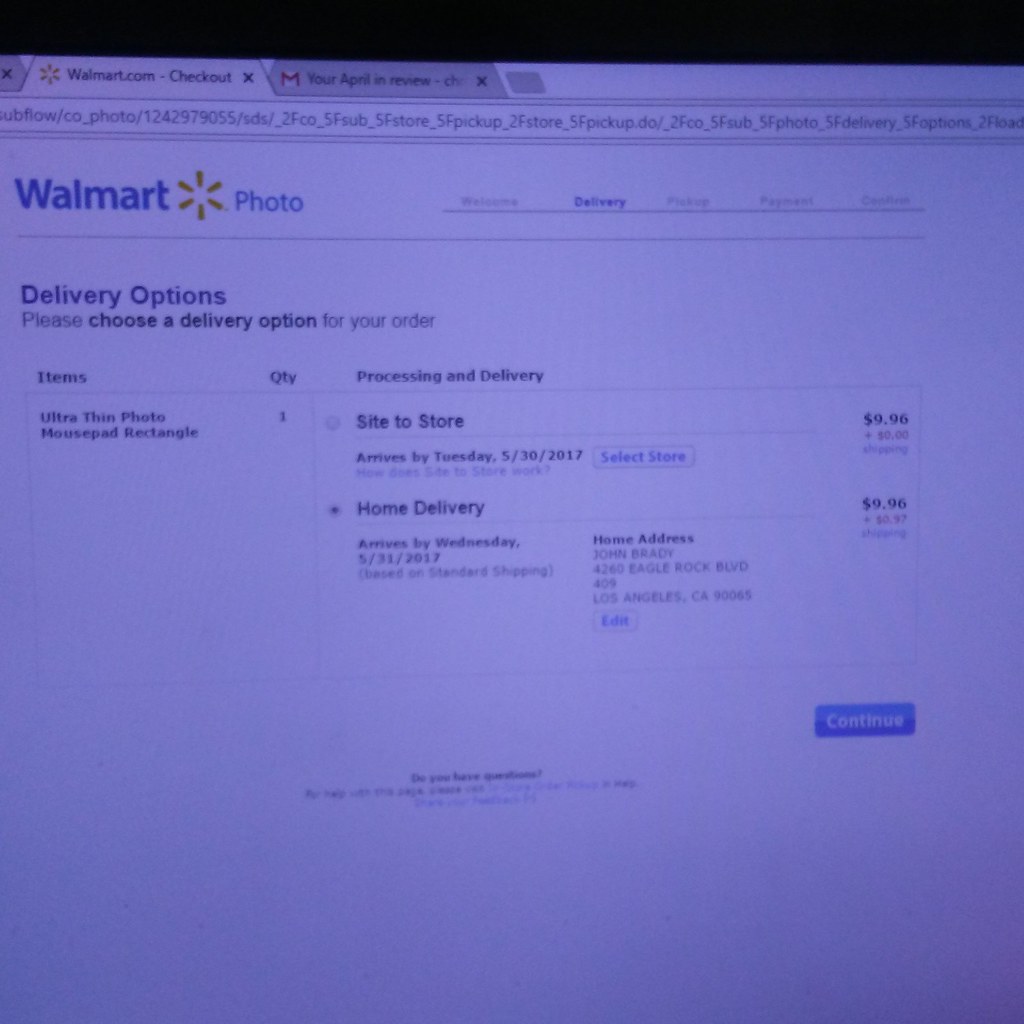The image is a color photograph of a computer screen displaying a Walmart.com checkout webpage. At the top, there is a black strip outside the screen, indicating poor lighting conditions, which also give the image a blue tint and a slightly blurry appearance. The browser shows two open tabs: an inactive Gmail tab in the middle, and an active Walmart.com tab with a long, illegible web address below it. The webpage itself is predominantly white with the blue Walmart logo and yellow star in the upper left corner, next to the word "photo" in blue.

Below this, in small black and blue text, there is an instruction: "Delivery options - Please choose a delivery option for your order." The options listed include site-to-store delivery and home delivery, with related addresses. Further down, the screenshot details the item being purchased: an "ultra thin photo mouse pad rectangle," priced at $9.96 for one quantity. In the bottom right corner of the webpage is a blue rectangle button with the word "Continue" written in white. The lower part of the image remains predominantly white and blank.